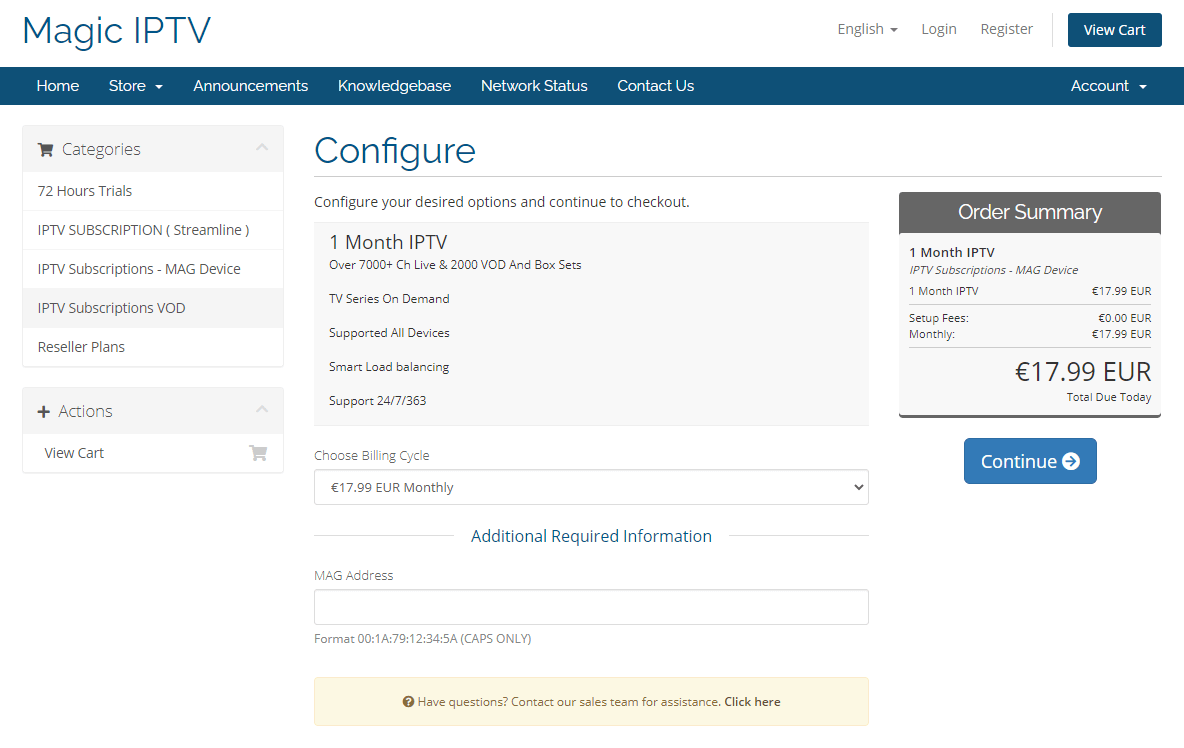The image is a detailed screenshot from the "Magic IPTV" website.

At the very top left corner, the website title "Magic IPTV" is prominently displayed. To the right, there is a language selection drop-down menu currently set to English, followed by buttons for "Login," "Register," and "View Cart."

Below this is a navigation bar with various sections: Home, Store (which includes a drop-down menu), Announcements, Knowledge Base, Network Status, Contact Us, and an Account drop-down on the right.

The main content of the page starts with a sidebar on the left titled "Categories." Listed under this are options including: 72 Hours Trials, IPTV Subscription Streamline, IPTV Subscriptions Mac Device, IPTV Subscriptions VOD, and Reseller Plans. The category "IPTV Subscriptions VOD" is currently selected.

The central body of the page details the selected category, starting with a section labeled "Configure Your Desired Options" and a "Continue to Checkout" button. It then lists the product specifics:
- One Month IPTV
- Over 7,000 Plus Channels Live
- 2,000 Video On Demand and Box Sets
- TV Series On Demand
- Supported on All Devices
- Smart Load Balancing
- 24/7/365 Support

Following this, the user is prompted to "Choose Billing Cycle," with a monthly fee of 17.99 Euro already selected. An "Additional Required Information" section asks for a "MAG Address," accompanied by a field for the user to enter this detail.

At the bottom of this section, it states, "Have Questions? Contact Our Sales Team for Assistance," with a clickable link for further help.

On the right side, a box labeled "Order Summary" recaps the order:
- One Month IPTV
- IPTV Subscriptions
- MAG Device
- One Month IPTV at 17.99 Euro
- Setup Fees: 0.00 Euro
- Monthly: 17.99 Euro
- Total Due Today: 17.99 Euro